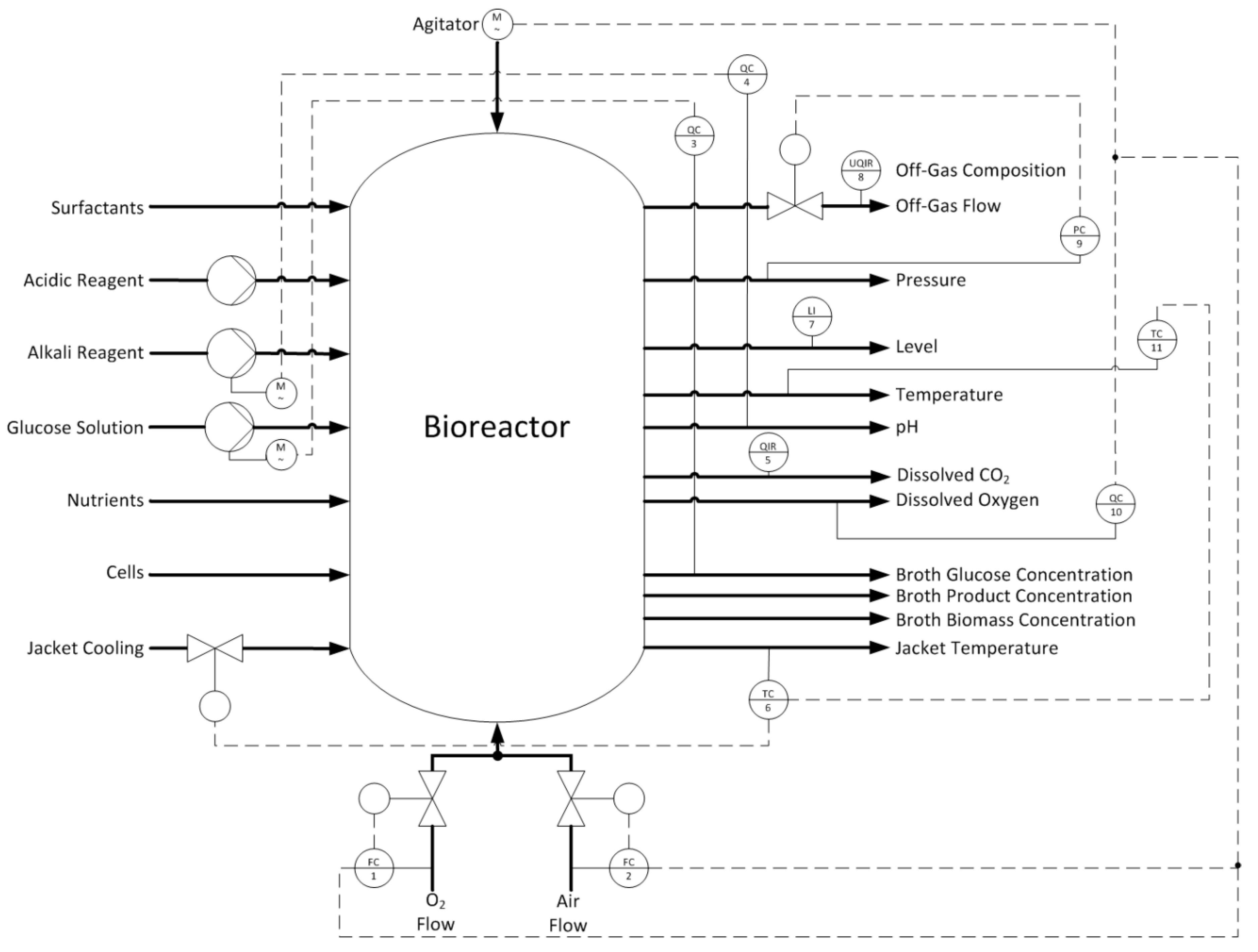The image is a detailed black-and-white diagram of a bioreactor, depicted with black text on a white background. At the center of the diagram is a large, pill-shaped oval labeled "bioreactor." Arrows and text descriptions surround this central shape, illustrating both inputs and outputs of the system.

At the top of the bioreactor, an arrow points downward and is labeled "agitator." Along the left side, arrows point from various inputs toward the bioreactor. These inputs include surfactants, acidic reagent, alkali reagent, glucose solution, nutrients, cells, and jacket cooling.

On the right side, arrows lead away from the bioreactor, indicating the outputs and parameters being monitored. These outputs and parameters include off gas composition, off gas flow, pressure, level, temperature, pH, dissolved CO2, dissolved oxygen, broth, glucose concentration, broth product concentration, broth biomass concentration, and jacket temperature.

Additionally, dotted lines connect various descriptions, and some descriptions are accompanied by circles with numbers or shapes, indicating further details or steps in the process. Altogether, the diagram comprehensively shows the inputs, outputs, and interconnections essential to the functioning of the bioreactor.